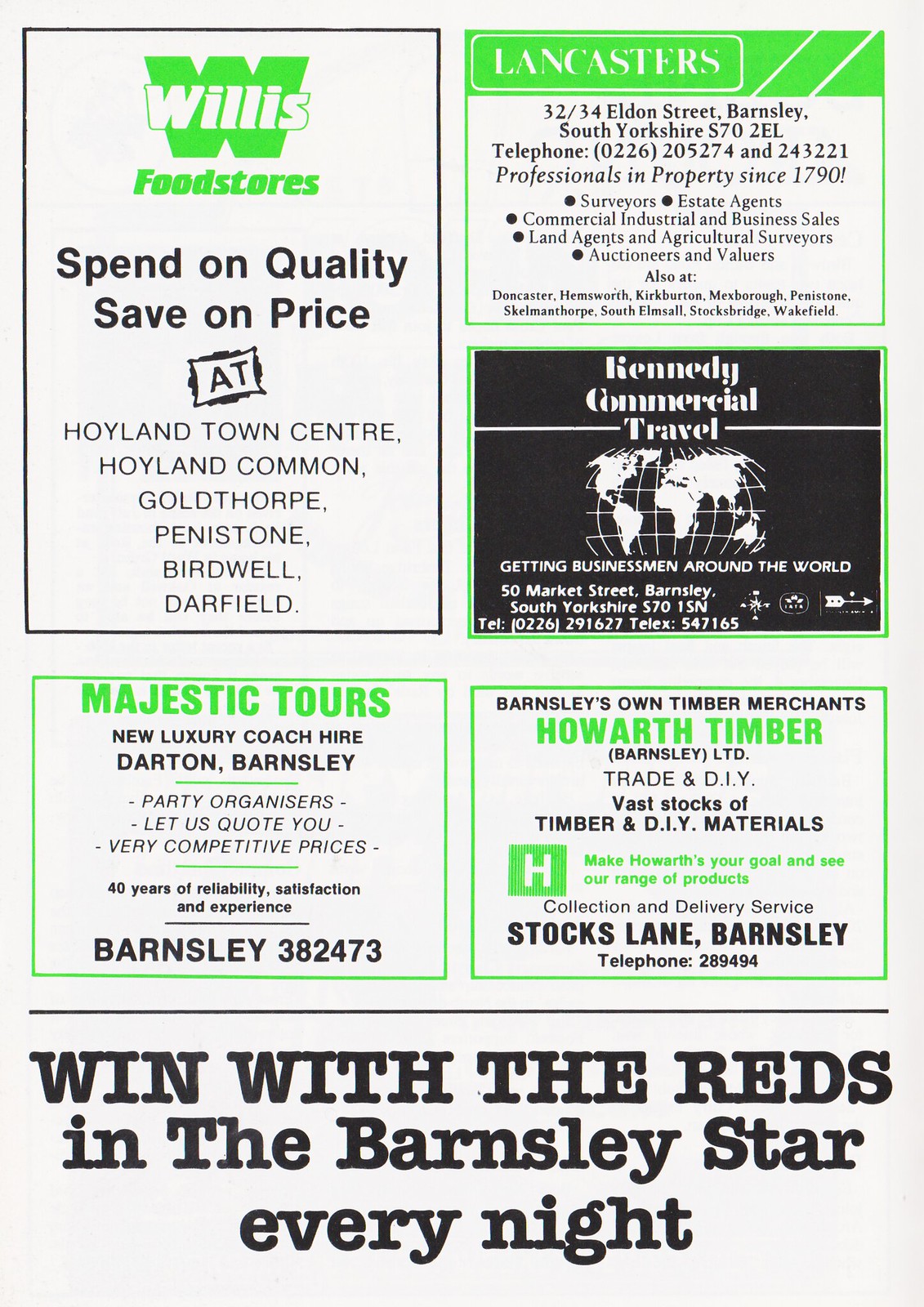This image is a page from a brochure, showcasing multiple advertisements on a white background with black text and bright green accents. At the very bottom, in black text, it says "Win with the Reds in the Barnsley Star every night."

On the left side, the upper corner features an advertisement for Willis Food Stores, with the slogan "Spend on quality, save on price." It lists locations in Hoyland Town Center, Hoyland Common, Goldthorpe, Pennistone, Birdwell, and Darfield. 

The right side, in the upper corner, holds an ad for Lancaster's on a green background. It provides detailed information including the address at 32/34 Eldon Street, Barnsley, South Yorkshire, S70 2EL, and two phone numbers: 0226-205274 and 243221. The ad emphasizes "Professionals and Properties since 1790" and mentions services like surveyors, estate agents, business sales, land agents, agricultural surveyors, auctioneers, and valuers.

In the center, there's an advertisement for Kennedy Commercial Travel, which touts "Getting businessmen around the world." It includes their address at 50 Market Street, Barnsley, South Yorkshire, S70 1SN, with phone number 0226-291627 and telex 547165.

On the bottom left side, there's an ad for Majestic Tours, promoting their "New Luxury Coach Hire" services from Darton, Barnsley. It mentions competitive pricing and lists the phone number Barnsley 382473.

On the bottom right side, the ad for Barnsley's own timber merchants, Howarth Timber, includes information about their timber and DIY materials, located on Stocks Lane, Barnsley, with a telephone number 289494.